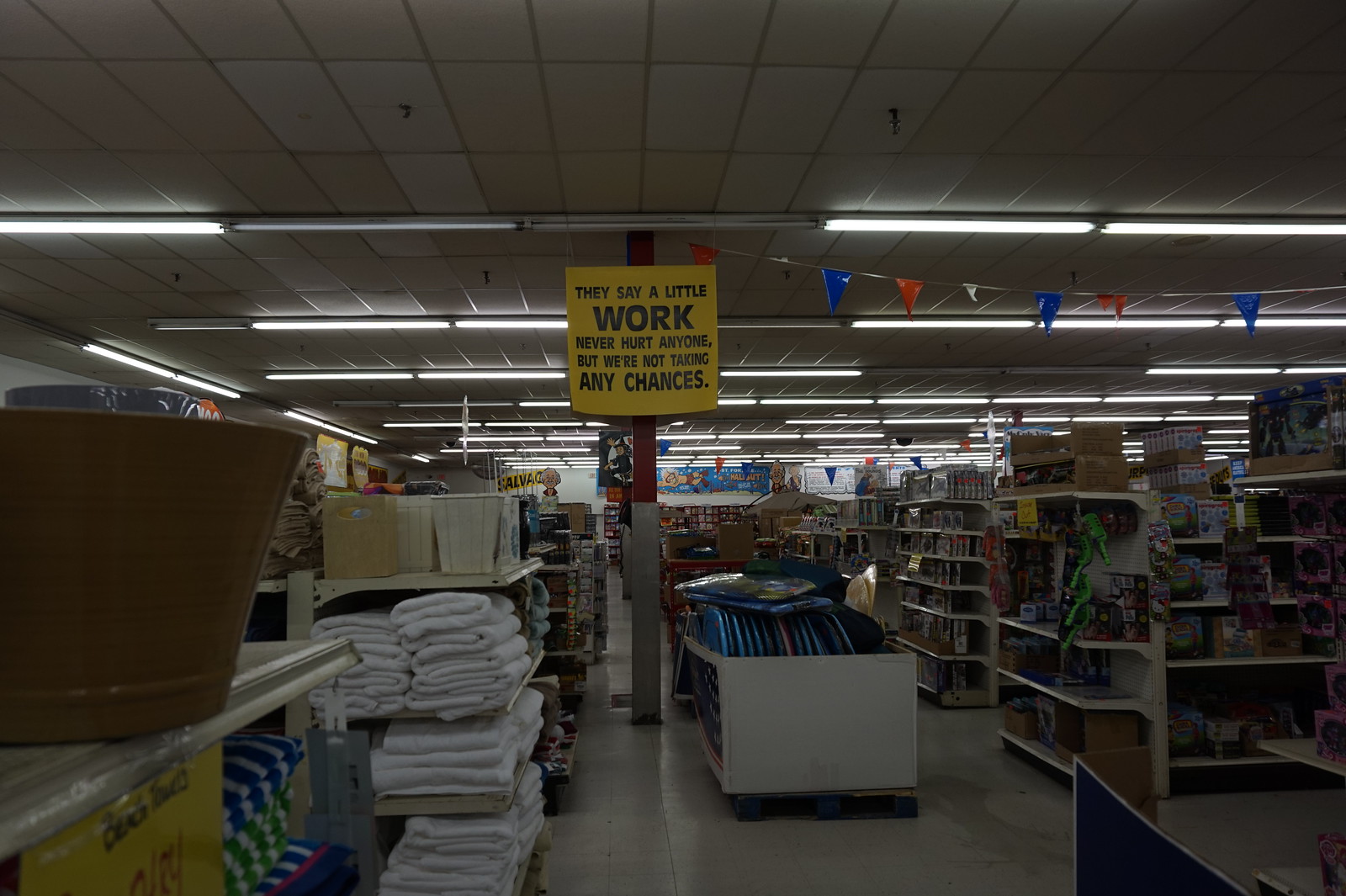This image captures the interior of a large hardware store, bustling with various sections and products. At the center, a prominent post stands tall with a red top and white bottom, displaying a whimsical message: "They say a little work never hurt anyone, but we're not taking any chances." The store is organized with aisles containing bins filled with miscellaneous items, including what appear to be boogie boards. On the left side, a metal shelf neatly holds a stack of folded towels, while the right side features a toy section. The overall decor of the store is accentuated by red and blue triangular flags strung across the ceiling, adding a touch of festivity. In the background, signs and a blue banner mark different areas, guiding customers through the expansive space.